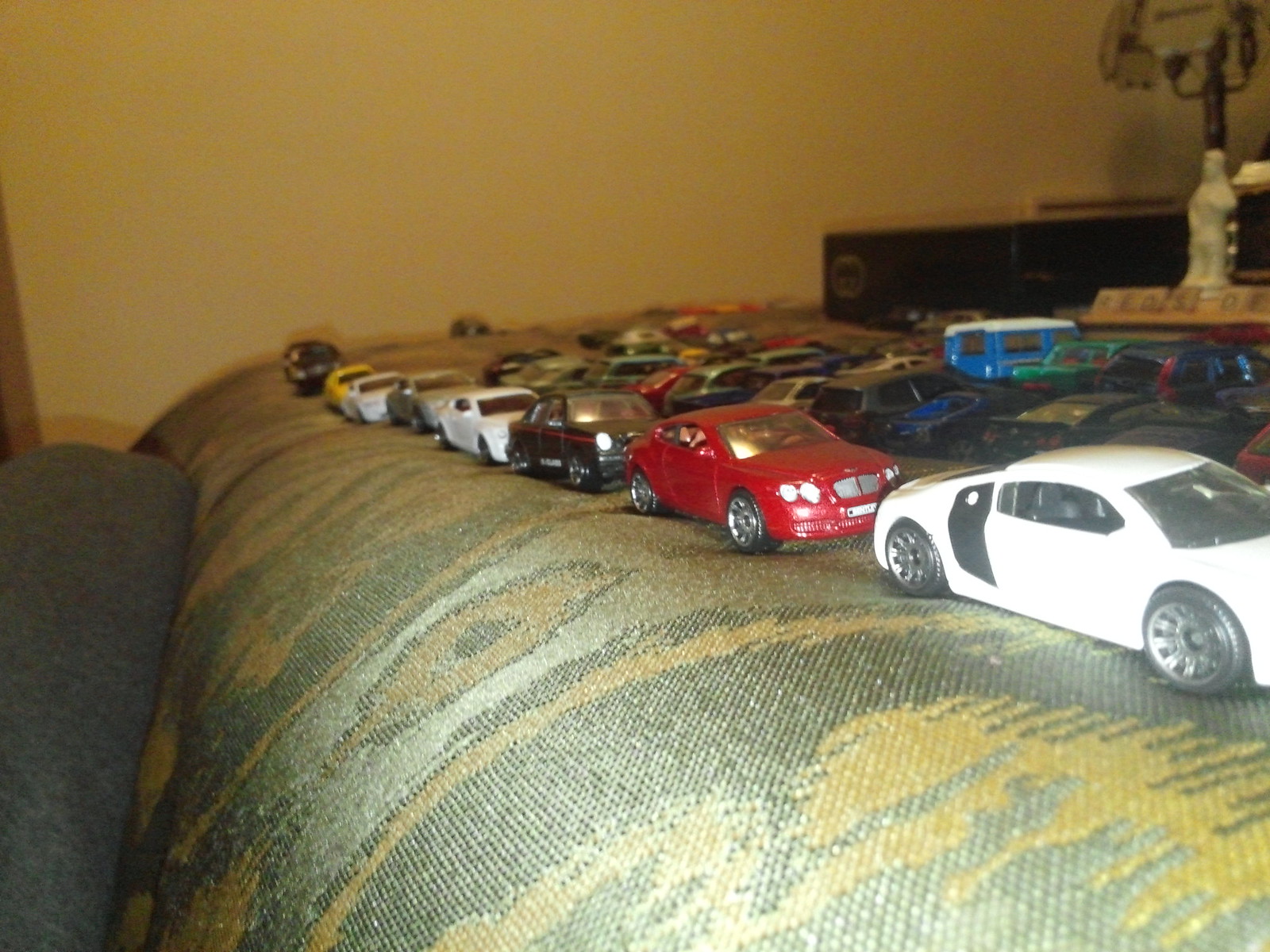The image depicts a vibrant collection of miniature cars, resembling Matchbox or Hot Wheels models, meticulously arranged in three rows atop a light brown piece of furniture with a shiny, yet muted stripy pattern of greens, yellows, and oranges. The cars are a mix of different designs and colors, including sedans, vans, and sporty cars in hues of white, black, red, silver, grey, green, and blue. The arrangement starts with a noticeable white and black car, approximately three inches long, followed by variously colored cars, with a distinctive tall blue van in the farthest row. In the background, a pale beige wall is partially visible along with a turned-off lamp with an old-style shade and a small decorative statue sitting on a black countertop. The setting suggests a cozy, lived-in space with a nostalgic, old-style ambiance.